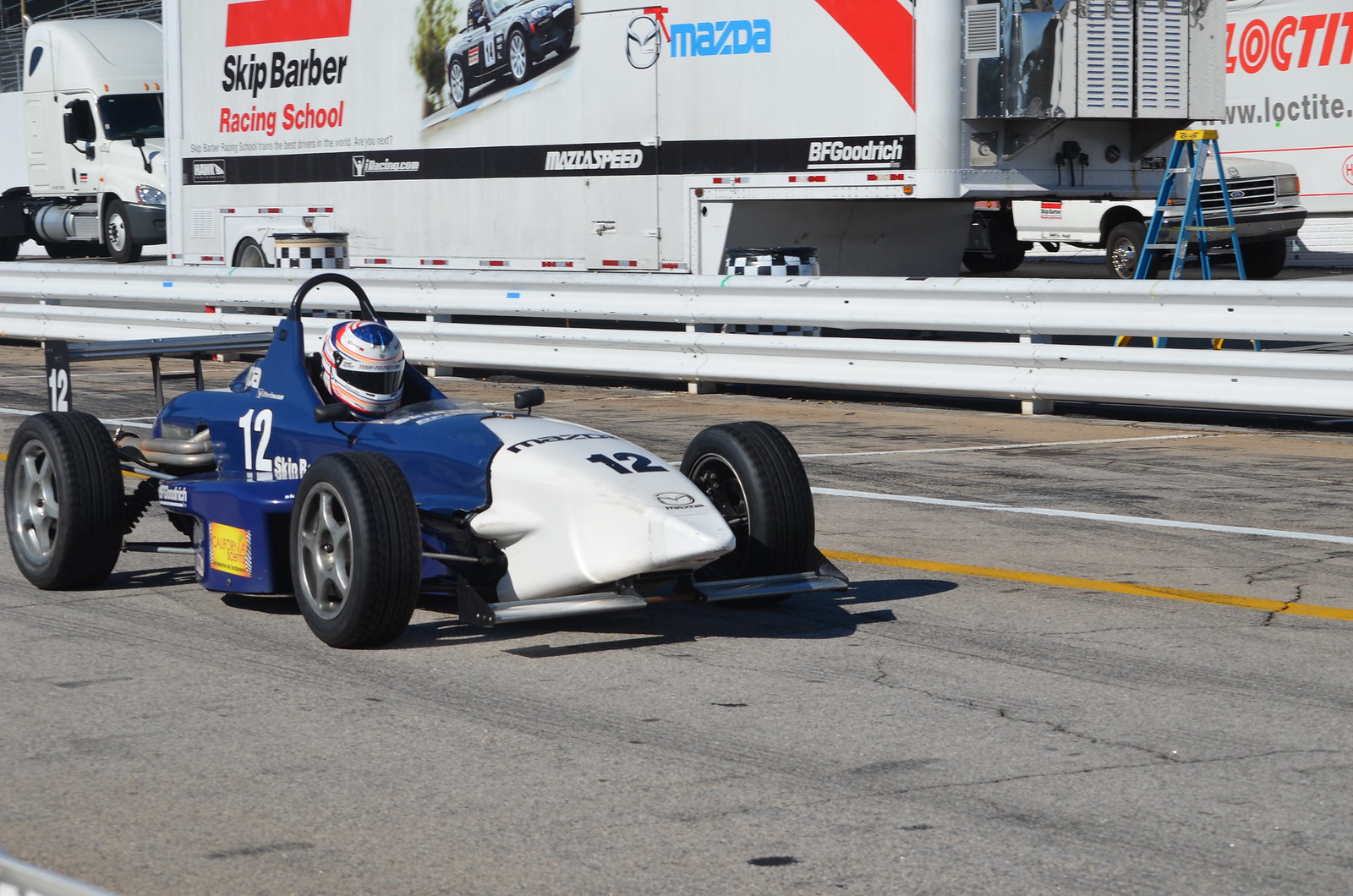The photograph features a small racing car, reminiscent of a junior Formula One car, with a compact body and a smaller wheelbase. The car sports a blue and white livery, with the front third painted white and the rear third in dark blue. Prominently displayed on the car is the number 12, indicating the driver's number, and a silver Mazda logo on the tip, signifying Mazda's sponsorship. The driver is equipped with a large racing helmet, reinforcing the car's purpose as a part of a racing event. 

The car is situated on a racing track, seemingly in a pit or staging area, possibly just coming off or heading onto the track. In the background, multiple white trucks and a large tractor-trailer are visible, the latter featuring the blue Mazda logo and branding for the Skip Barber Racing School. The trailer also has an image of a car and the school's name prominently displayed. A white guardrail runs parallel to the track, separating the racing area from the surrounding equipment and vehicles, adding to the professional race track setting.